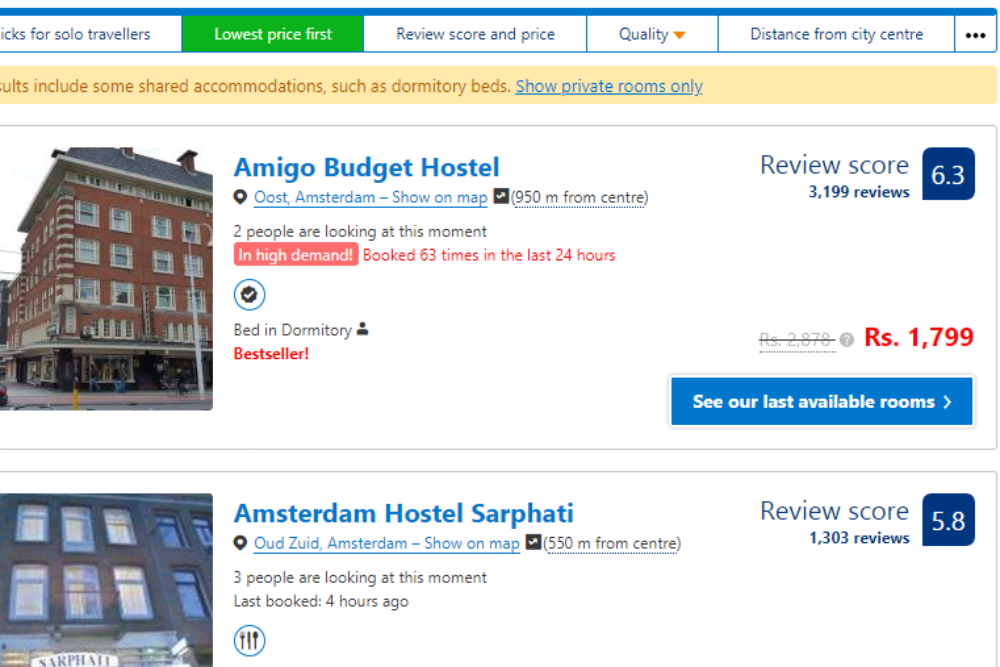This image is a screen capture from a web page with a white background. Featured prominently are two images of hotels located on the left side of the page. To the right of these images are detailed descriptions and ratings of the respective hotels.

At the very top of the webpage is a long rectangular navigation bar with various filtering options. The first option on the left is labeled "For solo travelers." Next to it, highlighted in green, is the option "Lowest price first." The following three options read "Review score and price," "Quality," and "Distance from city."

Beneath this navigation bar, the first hotel image appears. The hotel is a brown, four-story building. Beside the image, the hotel's name, "Amigo Budget Hostel," is displayed. Directly to the right of this name, a review score of 6.3 is visible, presented in white text within a blue square.